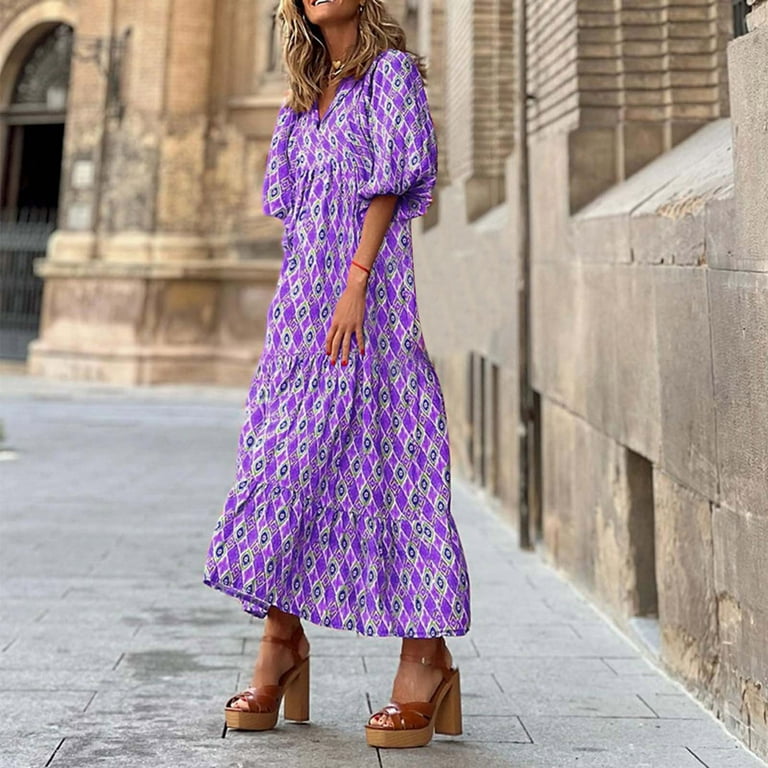In this image, a woman with long, blondish-brown hair is seen smiling, though the top part of her face is cut off above her teeth. She wears a flowing, ankle-length purple dress with a checkered pattern that includes green, blue, and white elements. The dress has loose, flouncy sleeves that end at her elbows and is styled like a caftan. Accessorizing her outfit, she sports a red bracelet on her wrist and her nails are painted red. She also has a gold necklace around her neck. On her feet, she wears brown leather platform sandals with chunky heels. The background suggests an old stone courtyard with a weathered, gray-tiled ground, evoking a possibly Italian setting. The stone building in the backdrop is in various shades of gray and light cream, with an open door visible on the left side of the image. The photograph appears to be a fashion marketing shot, perhaps reminiscent of the late 70s style.